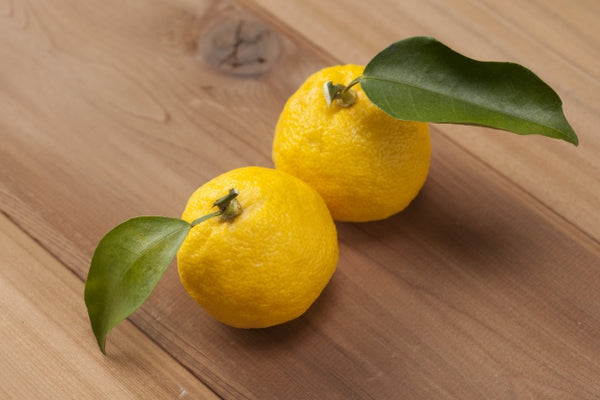This is a detailed photograph of two bright yellow lemons resting on a light brown wooden table, which features visible grain patterns and a large, cracked knot. Both medium-sized lemons are nearly perfectly round and positioned side by side, with one lemon slightly towards the bottom left corner and the other towards the bottom right middle. Each lemon has a small branch extending from the top, bearing a single, large, dark green leaf. The leaves are pristine and undamaged, with pointed tips and wide, smooth surfaces. The interplay of the vivid yellow lemons, the lush green leaves, and the rich, textured wood creates a striking visual contrast. There is no text present in the image.